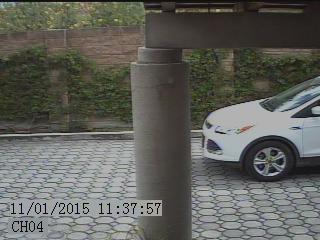The image is a camera footage screenshot taken outdoors, showing a parking lot on November 1, 2015, at 11:37:57 a.m. The scene features a central gray cement pillar with a circular pattern on the pavement leading towards it. On the right side of the image is the front half of a white car, which may either be stationary or in motion. The car is positioned facing left. In the background, there is a tan brick wall adorned with green ivy or foliage, which adds a touch of color to the otherwise gray and neutral-toned scene. The overall colors in the image include various shades of gray, white, green, reddish-brown, and some light brown, suggesting a daytime setting.